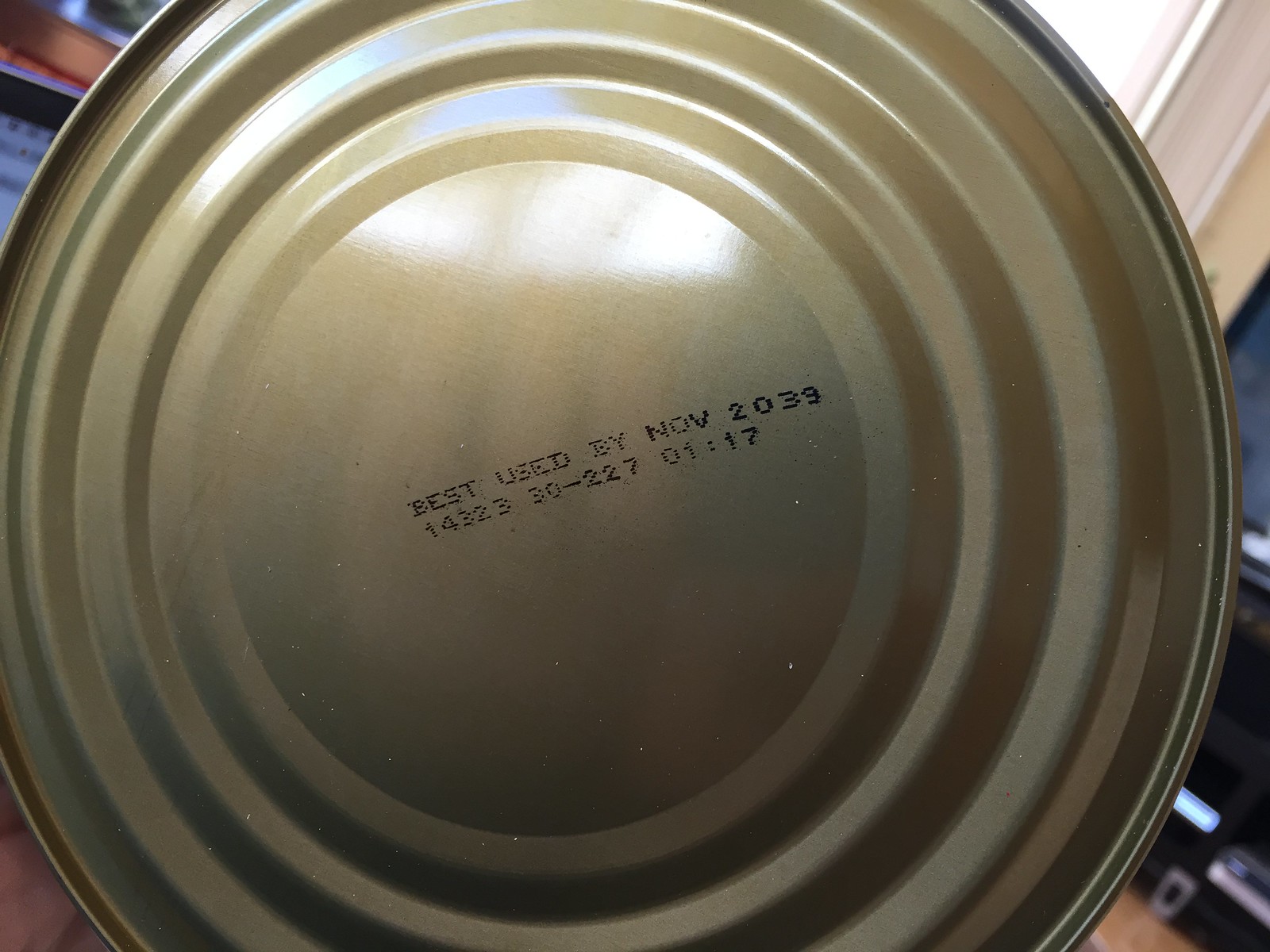The image depicts a silver can, showcasing what appears to be its top surface. Stamped on it are the details "Best used by November 2039" along with a code "142330-22701.17." The top view reveals concentric circles: one near the center and another closer to the edge. Light reflects subtly off the metallic surface, adding a sheen to the image.

In the background, the top right of the image shows a window through which natural light is streaming. Just to the right of the can, a TV is partially visible, though it's unclear whether it is powered on or off. At the bottom right, a wooden floor can be seen, adding a touch of warmth and contrast to the scene. The light source appears to be above and to the left, casting shadows on the lower part of the can and revealing tiny white specks of dust on its surface.